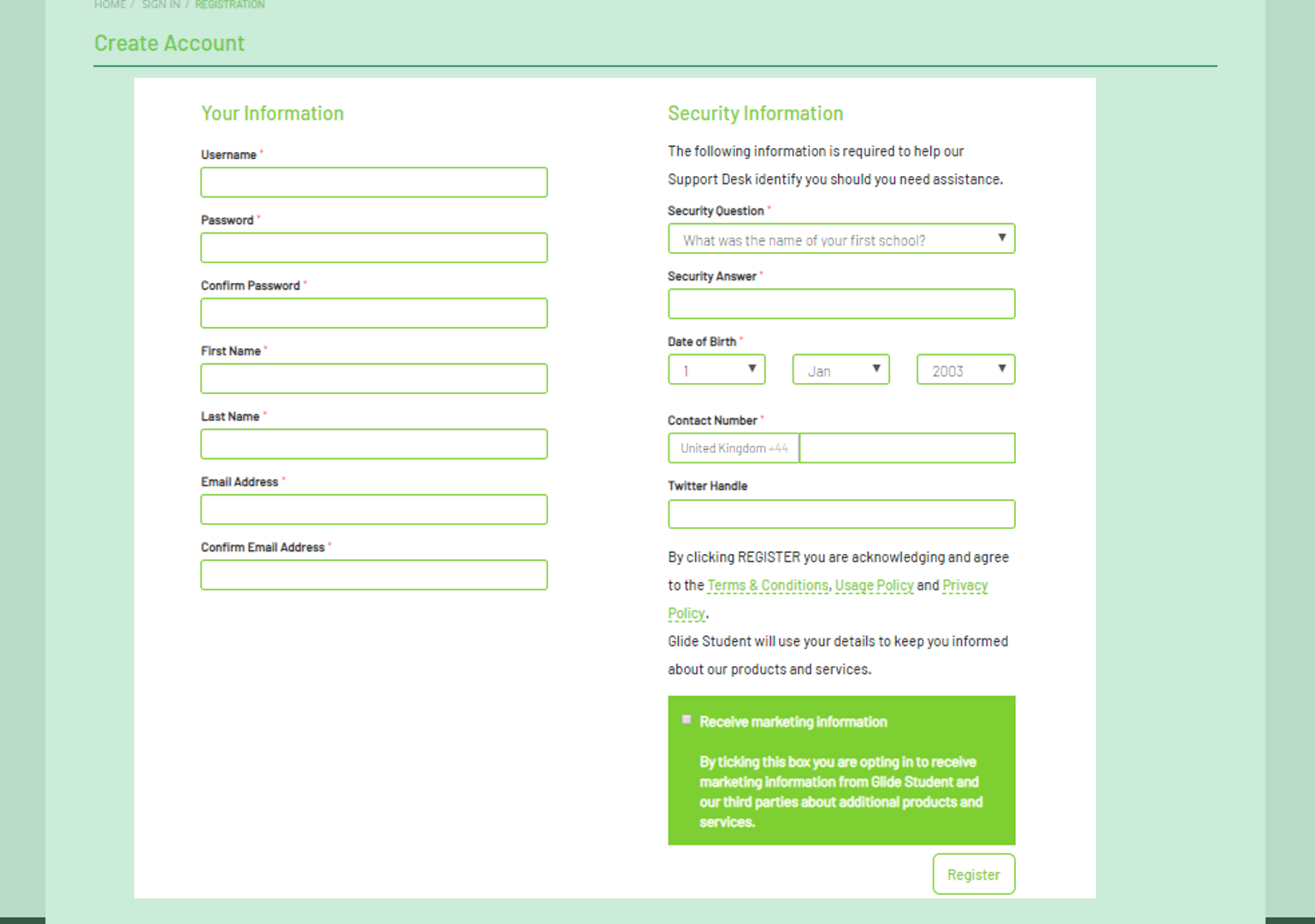The "Create Account" page predominantly features a lime green background, creating a vibrant and consistent color theme. The "Create Account" header itself is slightly off-color green, ensuring it stands out against the background.

In the top left corner, neatly aligned, are navigation options labeled "Home," "Sign-In," and "Registration," written in a contrasting color, which appears as a darker green, for easy visibility. The designer clearly favored the color green throughout the page.

Below the "Create Account" heading, the form begins with a section titled "Your Information." This section includes green-outlined input boxes with labels in black text. The required fields include:

- Username
- Password
- Confirm Password
- First Name
- Last Name
- Email Address
- Confirm Email Address

Each of these fields is marked with a small red asterisk, indicating mandatory completion.

On the right-hand side, there's a subsection titled "Security Information" in green text. Below this, a brief message in black text explains its purpose: "The following information is required to help our support desk identify you should you need assistance." This side includes further required fields:

- Security Question
- Security Answer
- Date of Birth (pre-filled as 1st January 2003)
- Contact Number (with a pre-filled country code of United Kingdom +44)
- Twitter Handle (optional)

At the bottom of the page, there's an important notice stating, "By clicking Register, you are acknowledging and agreeing to the Terms of Service, Use of Policy, and Privacy Policy. Glide Student will use your details to keep you informed about our products and services." 

There's also a green box with a checkmark option that says, "Receive marketing information," allowing users to opt-in to receive updates about additional products and services from Glide Student and third parties.

The form concludes with an action button at the bottom right-hand side. This button has a white background with a green outline and green text in the center that reads "Register."